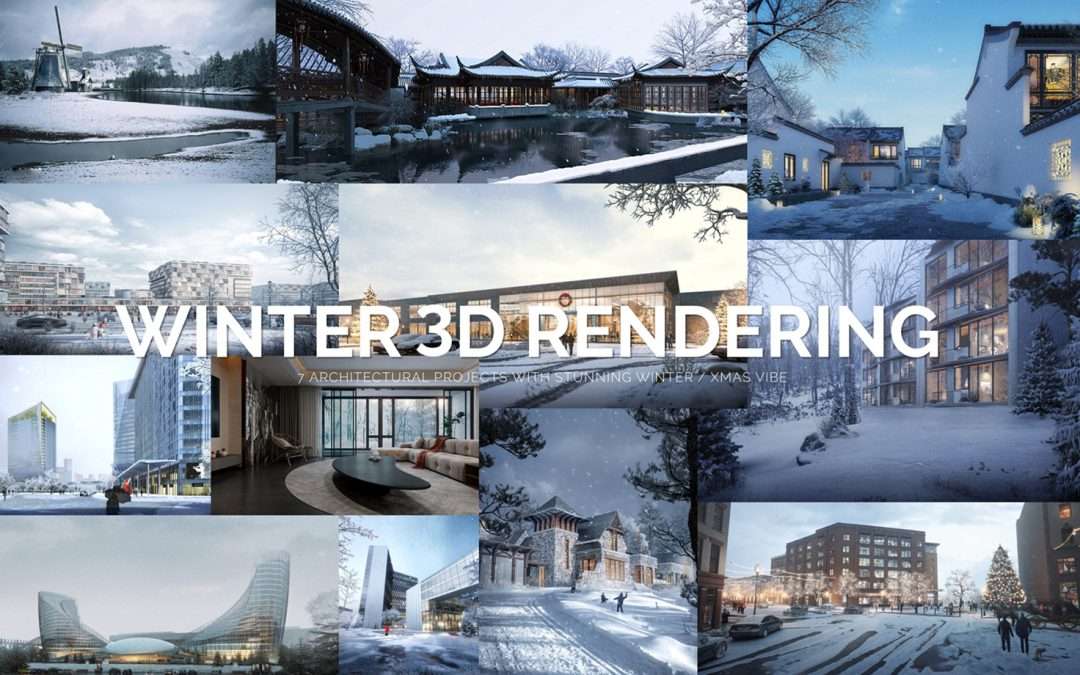The image is a wide horizontal compilation of highly detailed and realistic 3D renderings, comprising 16 panels depicting various winter cityscapes and landscapes. In the center, bold white text reads "WINTER 3D RENDERING," and it highlights "Seven architectural projects with stunning winter/Xmas vibes." 

Key scenes include:
1. A Japanese-style temple or palace complex featuring a lightly snow-covered wooden bridge over a man-made pond, gray skies, and leafless trees.
2. A U.S. cityscape with two men walking alongside a wintery roadside.
3. The top-most panels display what appears to be a winter resort or large gathering place, marked by an icy pond surrounded by snow.
4. On the right, a vertical stack of three images shows:
   - Single homes in a snowy setting.
   - Three-story suburban condominiums blanketed in snow.
   - A tall apartment building atop a snowy hill, with a snow-covered street and pedestrians.
5. Additional images portray various urban city scenes with tall buildings, all enveloped in a wintry climate, with snow covering the structures and streets.

This visually cohesive representation captures both serene and bustling aspects of winter environments, emphasizing architectural beauty amidst the snowfall.